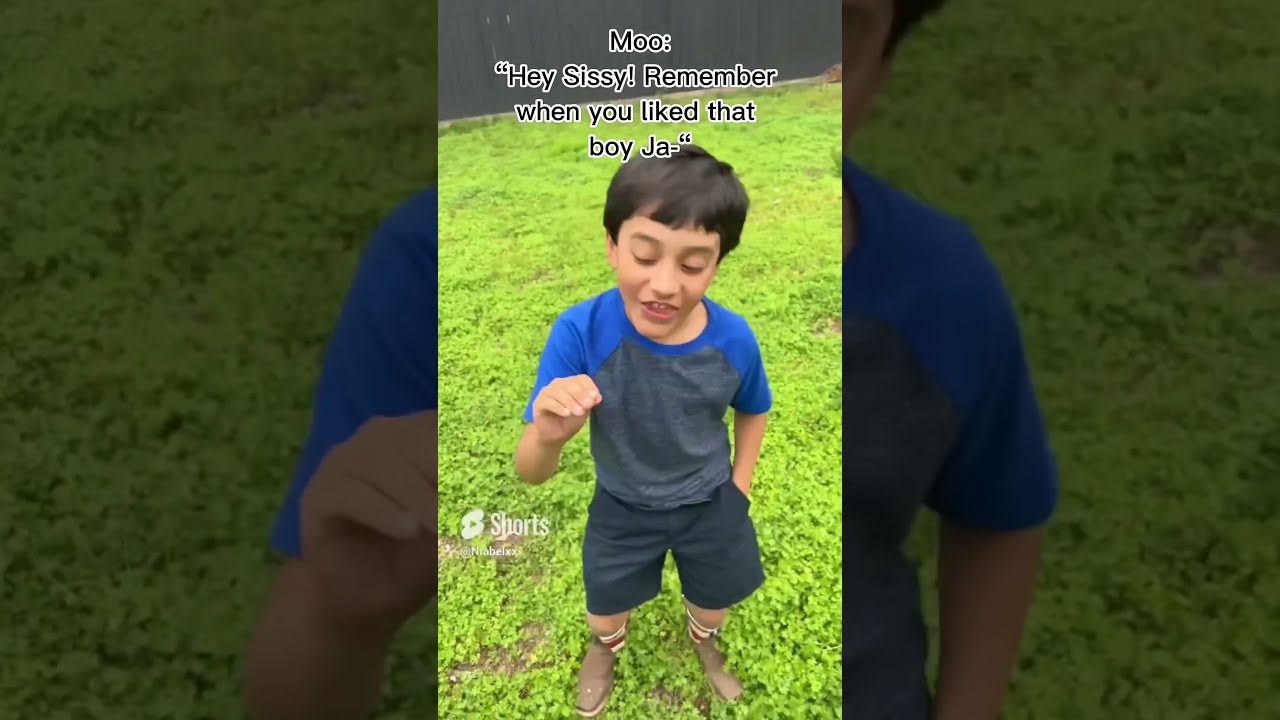In the image, a young boy, dressed in a blue and gray t-shirt, knee-length dark blue shorts, and brown boots with red and white trimmed tube socks, stands in the center of a grassy area, likely a backyard. His dark hair, styled in a bowl cut, frames his small smile as he playfully pinches his right hand, mimicking a puppet. His left hand rests in his pocket. A wooden fence, described as slate-colored, runs along the top of the image, providing a backdrop to the green grass and clover-like weeds below. The scene is captured as a YouTube Short, indicated by the YouTube Shorts logo, with a caption at the top reading, "Moo, hey sissy. Remember when you liked that boy? Ja."